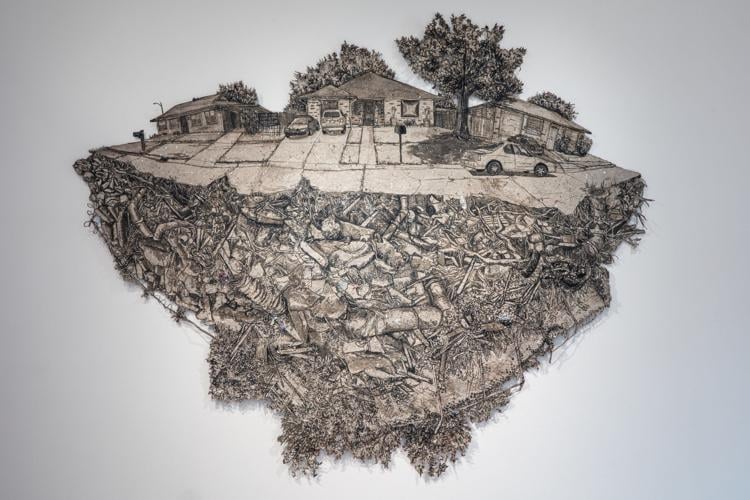The image depicts a meticulously detailed drawing, primarily in grays and shades of black, set against a pale background. It features three small, two-story suburban houses with pointed roofs, garages, and driveways. The house on the left is accompanied by a mailbox and a street light. The central house's driveway hosts both a car and a truck, while a dark car is parked in the driveway of the house on the right. A white car is seen parked by a tree in the foreground. The yards of the houses also include trees both beside and behind them. The scene presents a unique perspective showing what appears to be the slice of the earth beneath the street, revealing roots, rubble, and debris, giving it an illusion of the neighborhood segment floating on a chunk of land. The artistic style seems to mimic a stencil technique, combining the surreal with suburban tranquility.